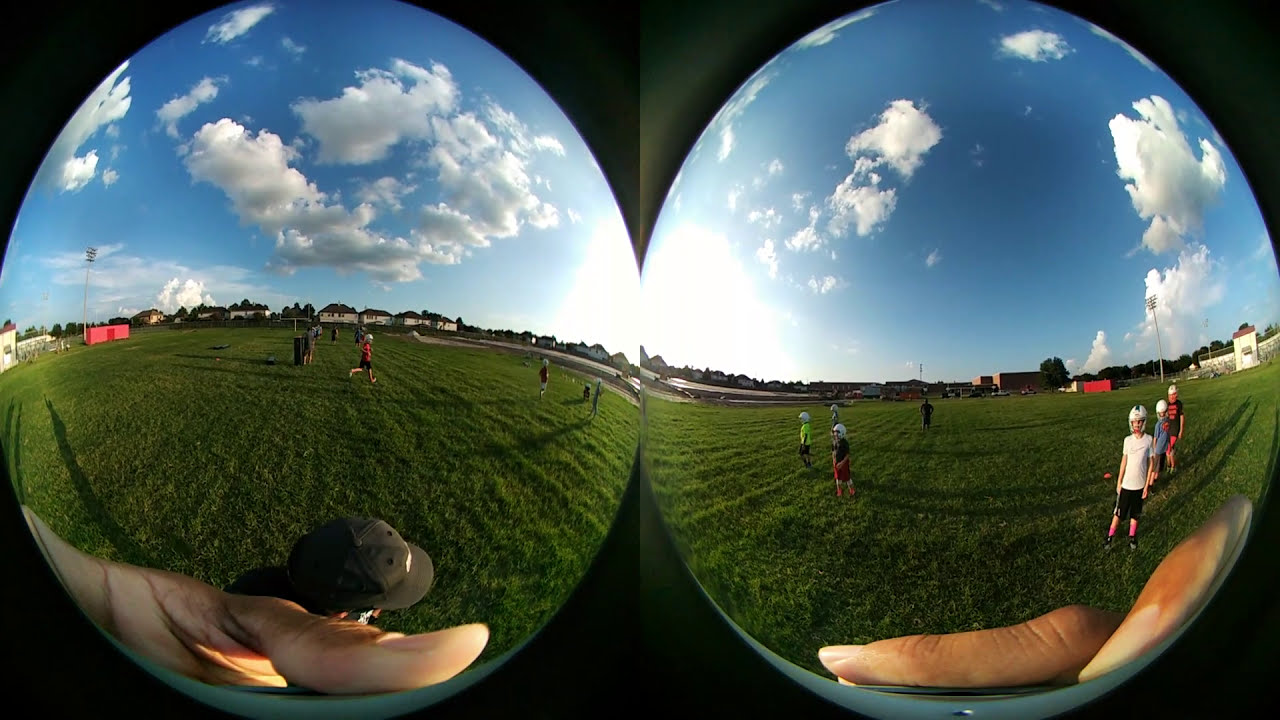The image showcases two adjacent fisheye lens views against a black background. Each circular view depicts a vivid scene of a youth football practice on a vast, green field under a bright blue sky peppered with white clouds. At the bottom of both circles, a person’s fingers and the top of their head, adorned with a black baseball cap, are visible, indicating they are holding the cameras to capture this scene.

The field is bustling with young players wearing white football helmets, t-shirts, and shorts. Some children are captured running, while others gaze curiously up at the cameras. The horizon reveals distant elements such as bleachers, a school building, storage lockers, and light poles—all integral to a typical football field setting. In the left image, a red structure is visible on the ground, and trees flank the scene. The right image mirrors much of the left but features slightly fewer clouds and more details of the buildings and kids in helmets, emphasizing the dynamic practice environment on this sunny day.